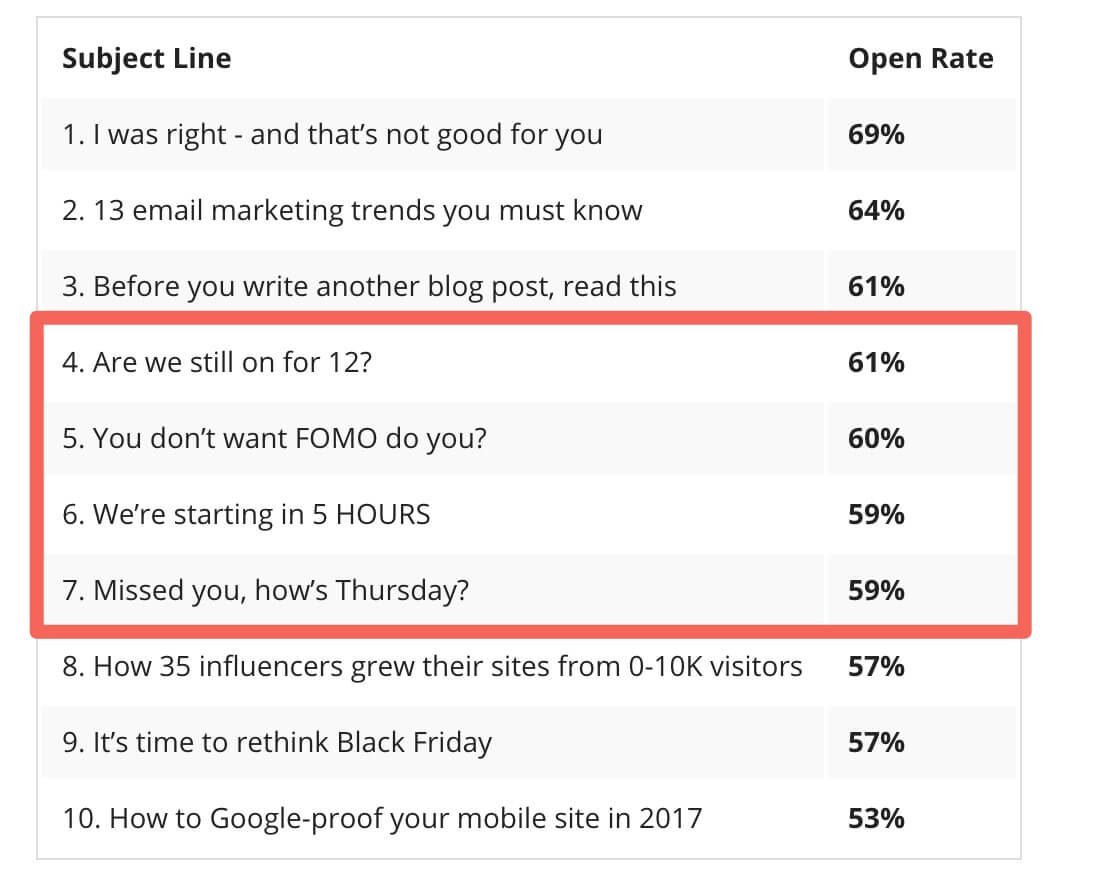The image is a detailed table with two primary columns titled "Subject Line" and "Open Rate," written in bold. The table is divided into horizontal rows listing various subject lines along with their respective open rates, expressed as percentages. 

The first column "Subject Line" lists these subjects:
1. I was right and that's not good for you
2. 13 email marketing trends you must know
3. Before you write another blog post, read this
4. Are we still on for 12?
5. You don't want FOMO, do you?
6. We're starting in five hours
7. Missed you, how's Thursday?
8. How 35 influencers grew their sites from 0 to 10,000 visitors
9. Time to rethink Black Friday
10. How to Google-proof your mobile sites in 2017

The second column "Open Rate" shows the corresponding percentages:
1. 69%
2. 64%
3. 61%
4. 61%
5. 60%
6. 59%
7. 59%
8. 57%
9. 57%
10. 53%

Rows 4 through 7 are highlighted within a red box, possibly indicating a specific categorization or emphasis. This table likely pertains to data for email marketing campaigns, showcasing different email subject lines and their effectiveness based on open rates. This could be valuable for online marketing strategies, reflecting consumer engagement with specific messaging.